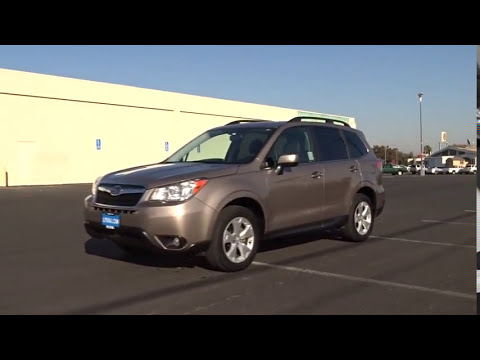The image features a slightly brownish-gray SUV, possibly a Ford or Toyota, with four doors and a hatchback, prominently parked in the foreground of a parking lot. This SUV, adorned with silver hubcaps and a removable blue tag on its front, is positioned against a beige-colored building with blue signs and a door, providing a clear focal point without surrounding cars to divert attention. The parking lot is paved with black asphalt and has white painted lines visible on the right side. In the background, a collection of cars—mostly white with one green vehicle—are dispersed around another building, which is accompanied by a long white fence stretching across the left part of the image. Light poles are strategically placed to illuminate the area at night. Above these elements, the sky forms the topmost layer of the composition.